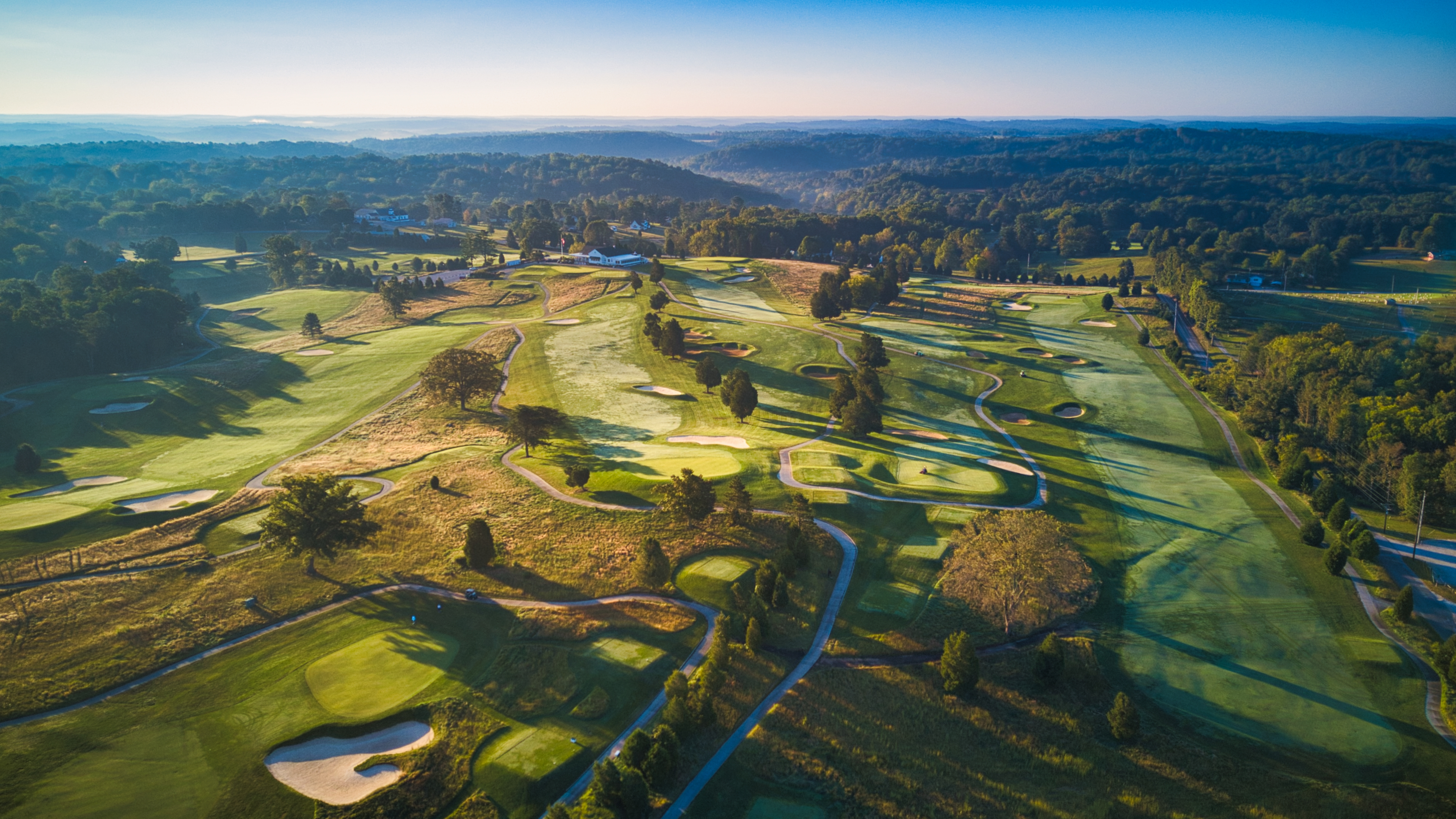This aerial photograph captures the expansive and meticulously manicured landscape of the Donald Ross course at the French Lick Resort. Taken during the late afternoon or early evening, the sun casts long shadows across the lush green fairways, verdant greens, and numerous sand traps. The course is surrounded by vast, rolling hills and dense forests that extend into the horizon, accentuating its serene, rural setting. Golf cart paths meander through the course, connecting the various holes. In the far distance, the clubhouse can be seen, accompanied by an empty parking lot and a flag waving next to it. The sky is a blend of blue and yellow hues, enhancing the picturesque quality of this beautifully maintained golf course. There are no players visible, adding to the tranquil ambiance of the image.